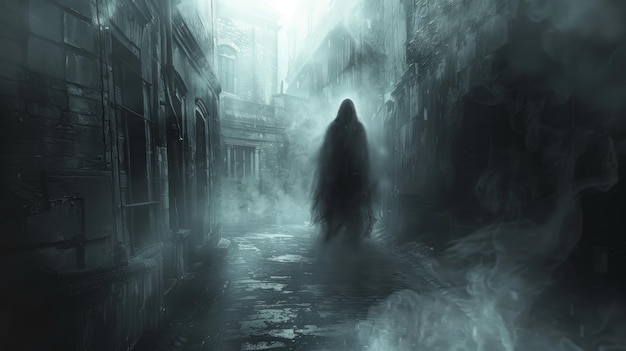This is an elongated, rectangular painting depicting a spooky, old-fashioned alleyway reminiscent of the 1700s. The scene is shrouded in mist and smoke, with a cobblestone road running through the center. Four blocky buildings frame the alley, two on either side and two visible in the background. In the middle of the alley stands a dark, cloaked figure, shrouded in mystery and almost ethereal with its gauzy, indistinguishable form. The figure's features are obscured, revealing only a vague silhouette that adds to the eerie atmosphere. The color palette is primarily composed of dark gray, light gray, black, and white, with touches of silver smoke, and a faint light emanating from the top middle of the painting, casting shadows that deepen the sense of unease. The painting, likely a mid-20th century digital art piece, captures the chilling essence of an ancient, mist-laden town, leaving viewers with a haunting impression of timeless mystery.